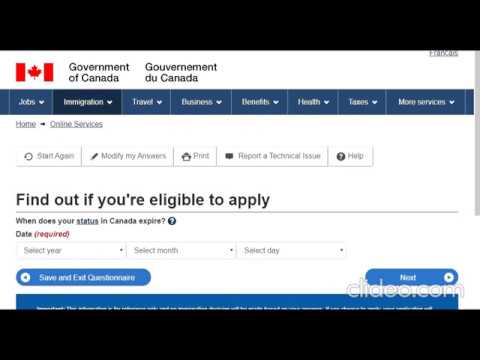The image depicts a government website with a white background. In the top left-hand corner, the text reads "Government of Canada," accompanied by the Canadian flag, which is white and red with a red maple leaf in the center. At the top of the page, there is a horizontal navigation bar with a dark blue background, featuring categories listed from left to right: Jobs, Immigration, Travel, Business, Benefits, Health, Taxes, and More Services.

In the main body of the website, centrally located, is a black text title that reads, "Find out if you're eligible to apply." This suggests the site offers information about eligibility for various government services, potentially including medical benefits, financial aid, job placement, or immigration services.

At the bottom of the page, on the right-hand side, there is a blue button labeled "Next" in white font. On the opposite side, the left-hand corner, there is another blue button labeled "Save and Exit Questionnaire."